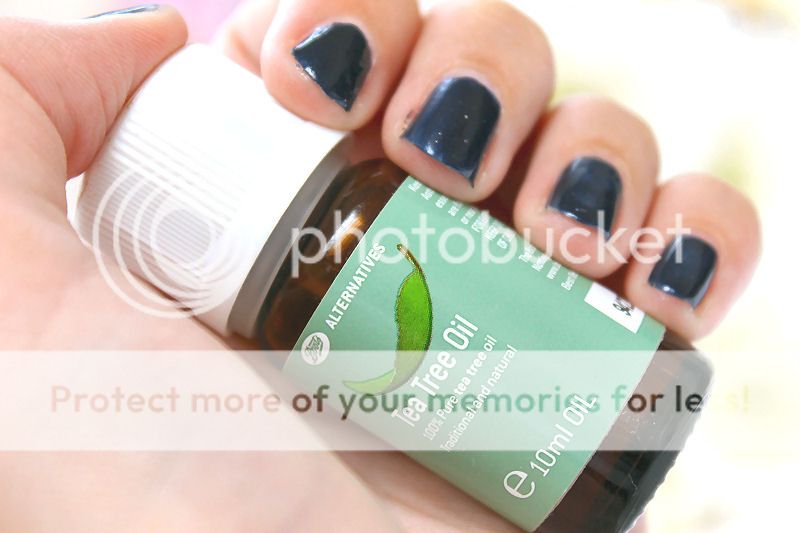The image features a woman's hand, with black-painted fingernails, holding a small, amber-colored bottle of tea tree oil. The bottle's label is light green, prominently displaying a bright green leaf that appears to be suspended in mid-air. The top of the label reads "Alternatives," and further down, it says "100% Pure Tea Tree Oil, Traditional and Natural." Below this text, there is the measurement "E 10 milliliters." The bottle is capped with a white, ridged screw cap. The woman's skin is light, and the background is bright, with hints of green and a touch of magenta near her thumb. A transparent watermark in white, saying "Protect more of your memories for less," overlays part of the image, indicating it's from Photobucket.